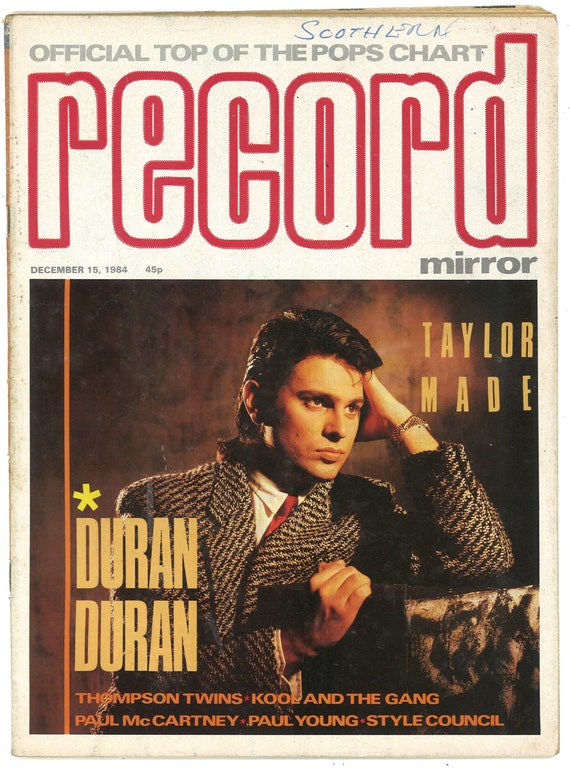The cover of the December 15th, 1984 issue of Record Mirror magazine prominently features the headline "Record" in large white letters outlined in red. Above this, in gray lettering on a white background, it reads "Official Top of the Pops Chart," with a handwritten note in blue ink that appears to say "Scoth Learn." Centered on the cover is a photograph of a man from Duran Duran, identified as either Duran Taylor or simply a member of the band, wearing a suit with multicolored gray and black lines. The man is captured in a casual pose, running his hand through his slick black, shoulder-length hair and leaning against a chair. A textured brown backdrop provides contrast to the image. Overlaid on the photograph in bright yellow letters is the name "Duran Duran." Below the main image, additional text mentions that this issue also features artists such as the Thompson Twins, Kool and the Gang, Paul McCartney, Paul Young, and Style Council.